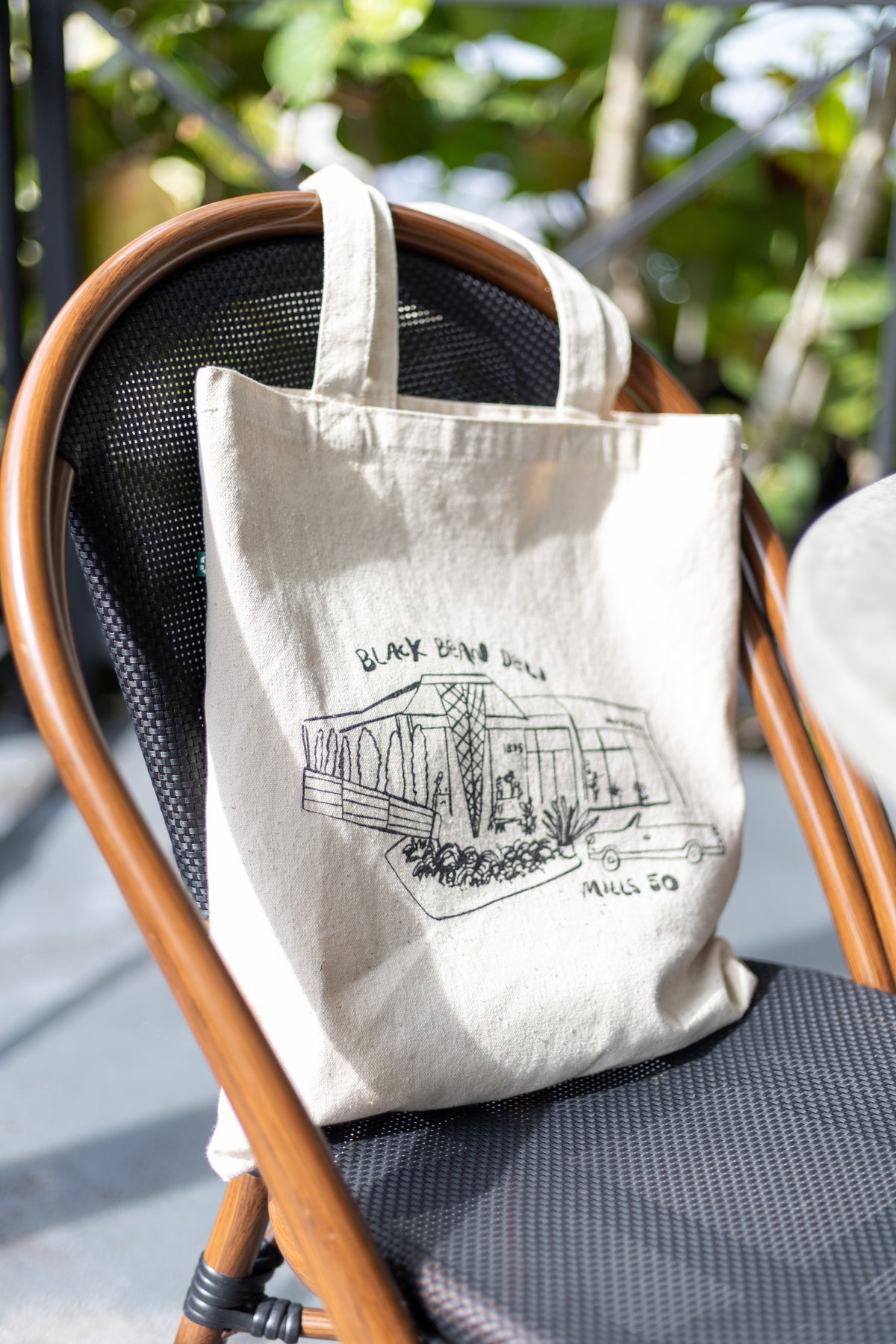The image captures a dark wooden chair with a round shape and cane mesh back and seat, situated on a porch. Draped over the back of the chair is an off-white reusable canvas shopping bag with two straps. The bag features a black-and-white illustration of a store, with text that reads "Mills 50" at the bottom and a depiction of trees, shrubs, and windows. The background, rendered in a bokeh effect, includes blurry elements of rain, leaves, flowers, bushes, and a light railing, along with the edge of a round white table. The setting appears to be outdoors, giving the scene a cozy, natural atmosphere.